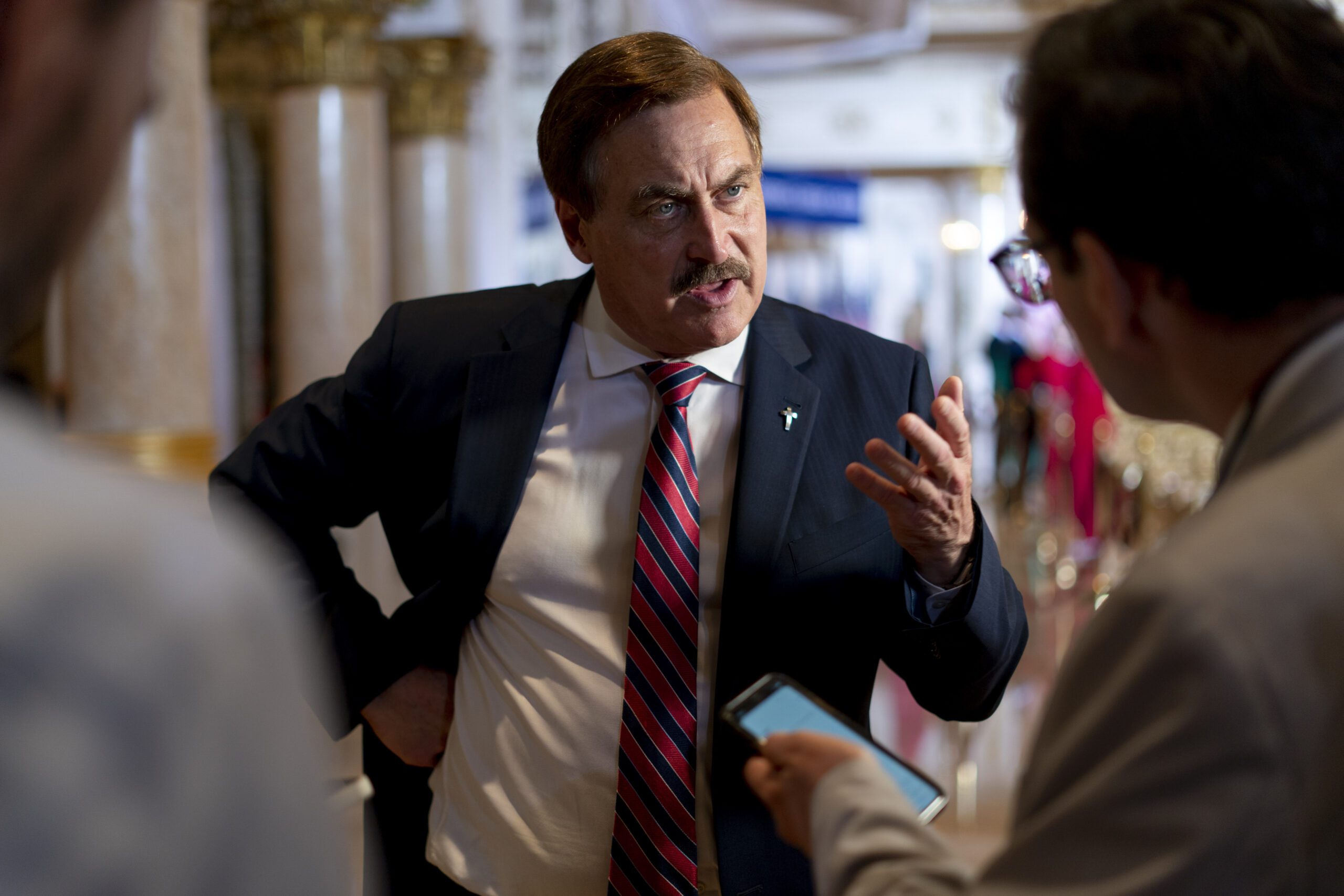In this detailed photograph, Mike Lindell, the CEO of MyPillow turned conspiracy theorist, is seen in a formal setting that appears to be a grandiose property, possibly linked to Donald Trump, given the opulent gold and marble columns in the background. Lindell is dressed in a dark blue or black suit jacket, accented with a small silver cross pinned to the right side. His attire includes a crisp white button-down shirt and a blue and red diagonally striped tie. He sports his characteristic brown hair and mustache. 

Lindell’s stance is confident: one hand rests on his hip, slightly pulling back his jacket to expose his white shirt beneath, and his other hand is raised to his mouth while he appears to be speaking or gesticulating towards another man, whose back of the head is visible. This man seems to be showing Lindell something on an iPhone, possibly recording or sharing information. The scene has the air of a serious discussion, potentially involving political matters or a press interview, bathed in the authoritative ambiance of a grand setting marked by large, luxurious pillars.